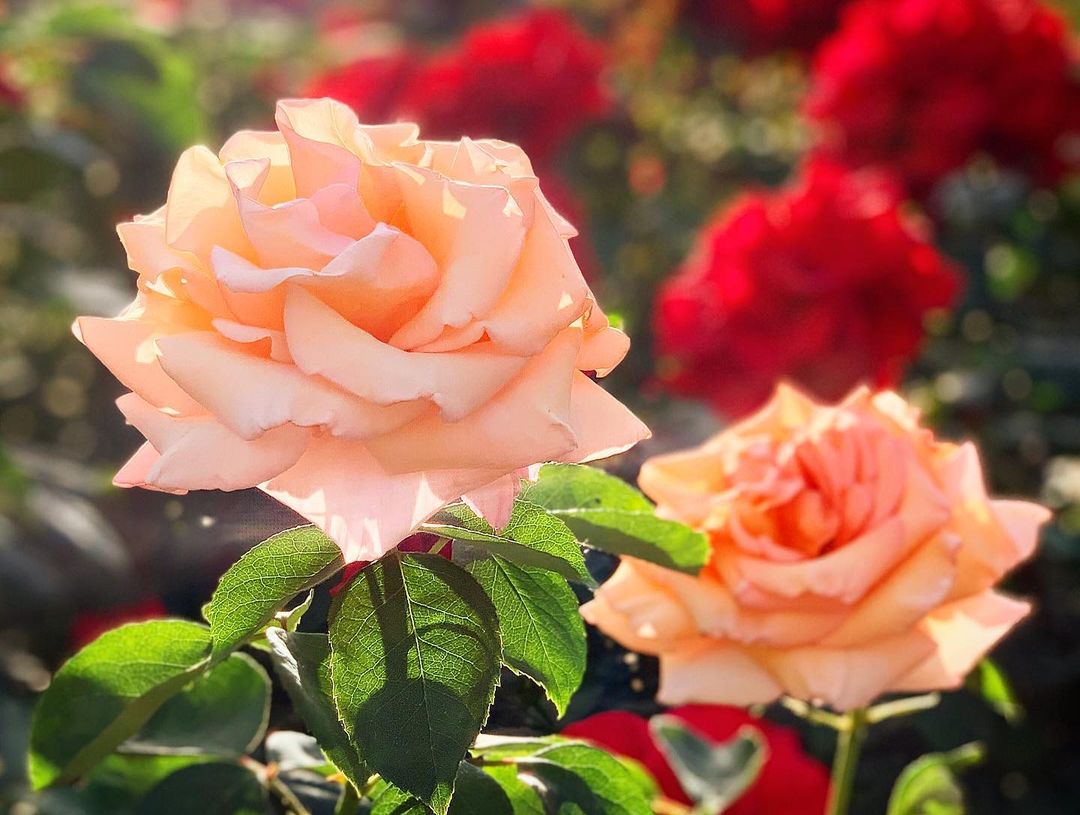The image captures an exquisite outdoor scene during the day, featuring the vivid and radiant colors of blooming flowers. Dominating the foreground are two beautifully blossoming pink roses, positioned with the larger and fuller one on the upper left and the smaller one on the bottom right. These delicate roses showcase light, almost translucent green leaves beneath them, which catch the sunlight, giving an effect of subtle shadows and highlighting the thinness of the leaves. In the background, slightly blurred to enhance the depth of the image, are striking red roses, also in full bloom. The sunlight reflecting off the petals and leaves adds a bright, almost luminous quality to the overall scene, emphasizing the vivid contrast of pink, red, and various shades of green. The photograph, with its meticulous details and play of light and shadow, creates a captivating portrayal of these flowers bathed in daylight.